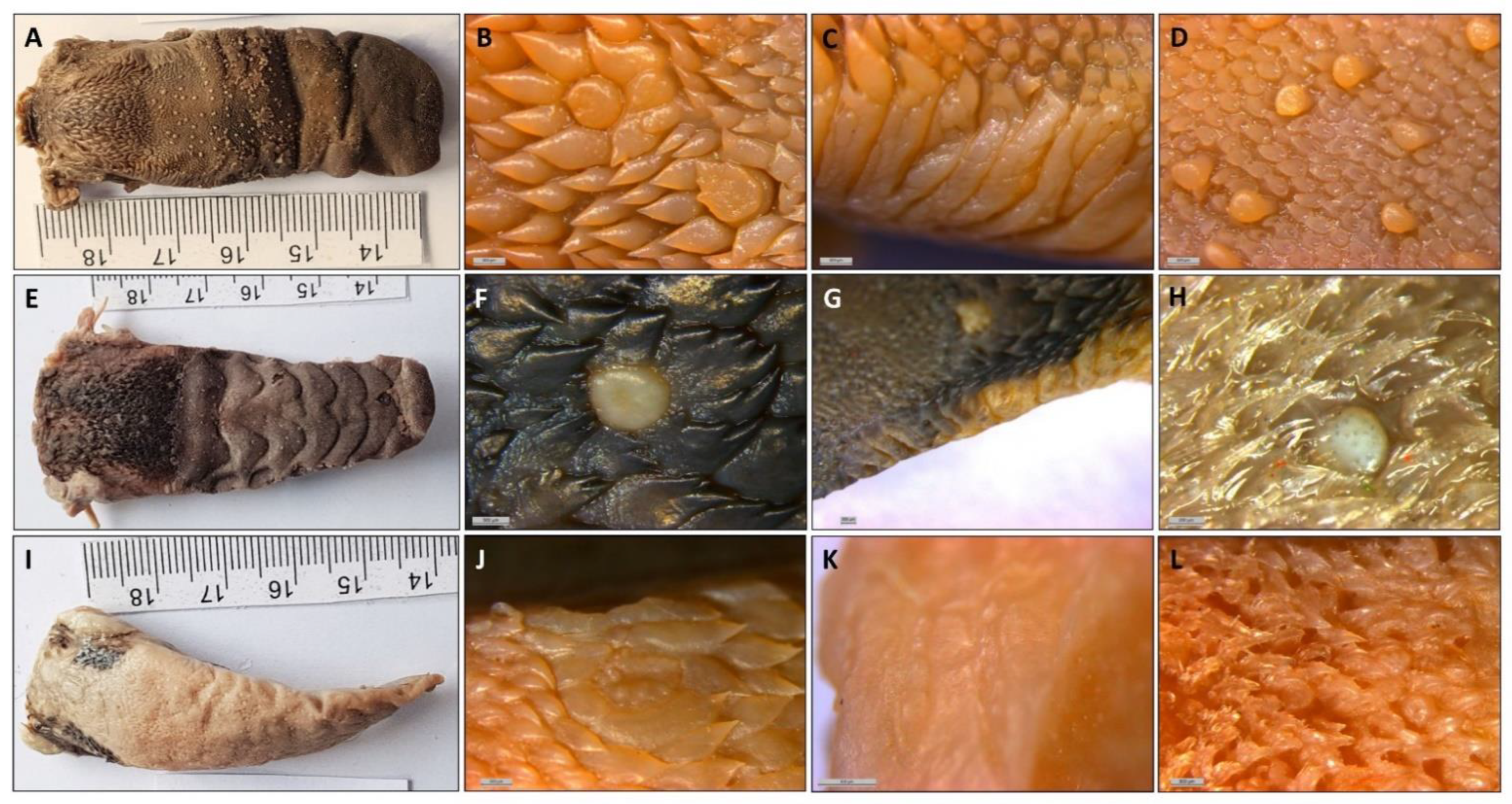The image consists of 12 small photographs arranged in a 4 x 3 grid, capturing an extreme close-up study of an unidentifiable organism. In the leftmost column, labeled A, there are three sequential photographs of what appears to be the same organism, possibly a larva, worm, or some kind of parasite, each alongside a small tape measure showing it to be approximately 5 centimeters in length. The top photo depicts a rough, brown exterior. The middle image shows a somewhat furry brown segment with defined sections. The bottom photo reveals a white, shriveled form with only a few brown patches, suggesting the organism might be dead.

The remaining nine photographs on the right display extreme close-ups of the organism’s texture and surface, capturing peculiar details. The top row reveals mottled, pulpy areas reminiscent of an orange's surface. The two central images in the middle row are darker, stained, and have white pustules, possibly indicating disease. The final row showcases more dramatic close-ups, including golden tendrils or hair-like structures. These detailed images suggest a focus on various stages of the organism's life cycle and its unique textures and features, presenting a bizarre and somewhat unsettling study of the unknown entity.